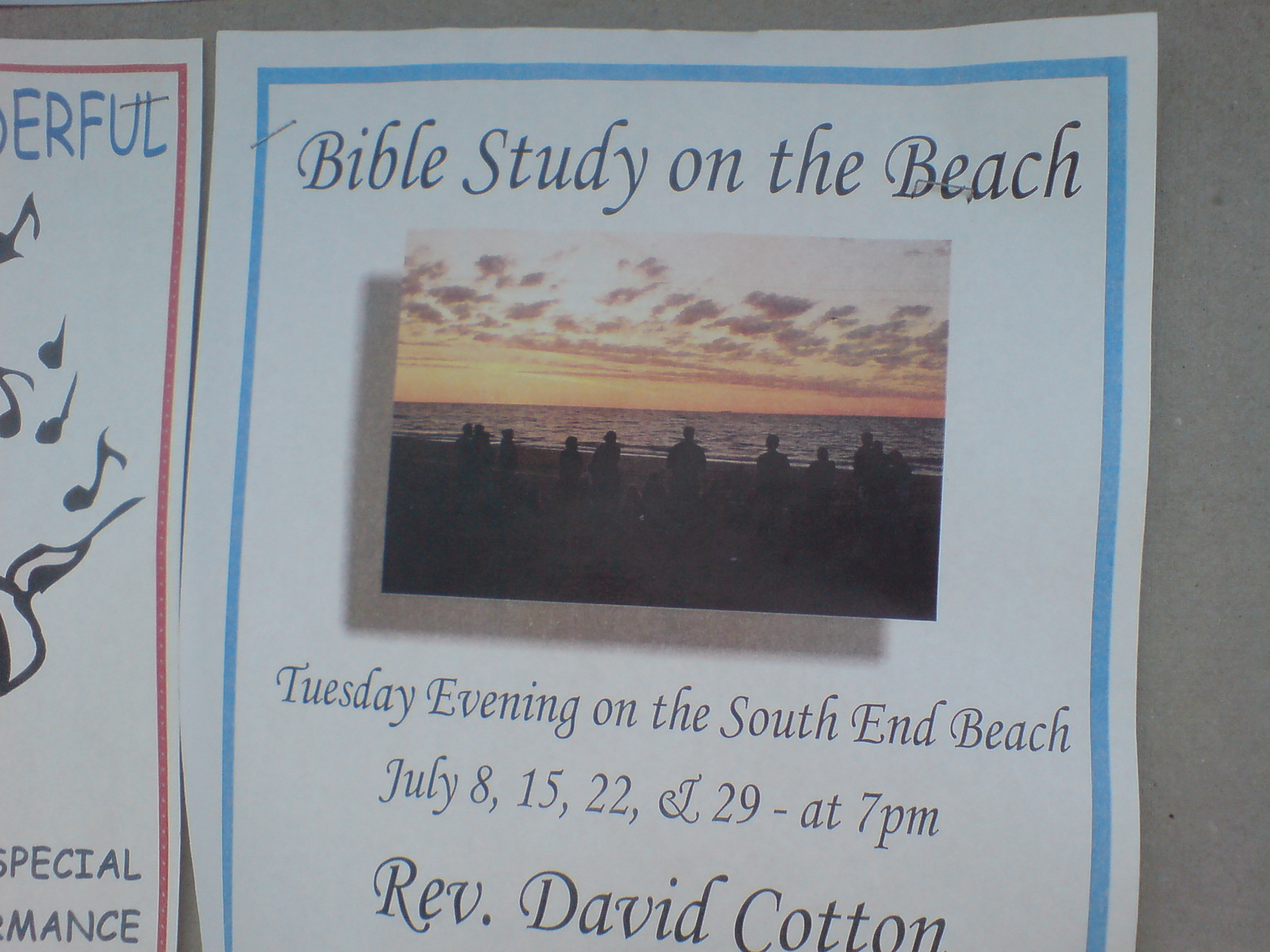In the image, there is a single, prominently displayed flyer centered against a gray wall or background. The flyer is bordered with a rectangular light blue frame and features a detailed event advertisement. At the top, bold text reads "Bible Study on the Beach." Below this heading is a photograph depicting silhouettes of a small group of people gathered on a beach at sunset. The sky is tinged with shades of orange, reflecting off the waters in the background, and a few clouds are visible, contributing to the serene twilight atmosphere.

Beneath the photograph, the flyer details the event schedule, stating, "Tuesday evening on the South End Beach, July 8th, 15th, 22nd, and 29th at 7 p.m." Further down, at the bottom of the flyer, it lists "Rev. David Cotton" as the organizer or leader of the event. 

Additionally, to the left of this main flyer, there is a glimpse of another flyer distinguished by a red border. This secondary flyer features some music notes and partially visible text, though specific details are indiscernible due to it being cut off in the image. The color palette of the entire scene includes shades of gray, white, red, light blue, orange, and black. The overall appearance and layout suggest this is an advertisement for an upcoming series of events suitable for those interested in Bible study sessions on the beach during sunset.